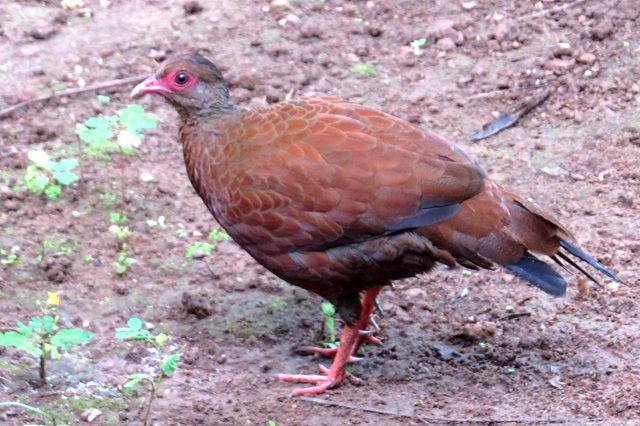The image depicts a brownish bird, likely a chicken, standing on a dirt surface outdoors. The bird is centrally positioned in the photograph and has distinct features such as a yellowish beak, peach or pinkish feet, and a few sharp spurs on the back of each leg. It has pinkish skin around the eyes extending to the beak. The tail feathers are dark gray, and there are touches of gray on the back of its head. The background is predominantly a dirt ground with sparse green plants and weeds showing through. The scene includes a variety of colors, primarily different shades of brown, tan, and green, with some touches of red and black. This outdoor setting is captured with a focus on the bird, which is not a rooster but closely resembles a chicken, against a natural, earthy backdrop.